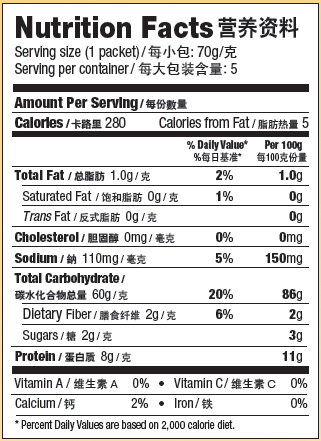This photograph captures a detailed view of a nutrition facts label. The label is predominantly white with black text and is bordered by very thin black and yellow lines. At the top, "Nutrition Facts" is prominently displayed in black font, accompanied by several Asian characters. Below, the label specifies the serving size as "one packet," followed by more Asian characters, and notes that there are five servings per container. 

The nutritional breakdown includes: 
- Calories: 280
- Calories from Fat: 1
- Total Fat: 1g
- Saturated Fat: 0g
- Trans Fat: 0g
- Cholesterol: 0mg
- Sodium: 110mg
- Total Carbohydrates: 60g
- Dietary Fiber: 2g
- Sugars: 2g
- Protein: 8g

Additionally, the percentages for daily values indicate:
- Vitamin A: 0%
- Calcium: 2%
- Vitamin C: 0%
- Iron: 0%

At the bottom, a note reads that the percent daily values are based on a 2,000 calorie diet. Asian characters follow each nutritional category, providing the names and measurements in grams and percentages. The overall layout and design adhere to a clear and structured format to ensure easy readability.